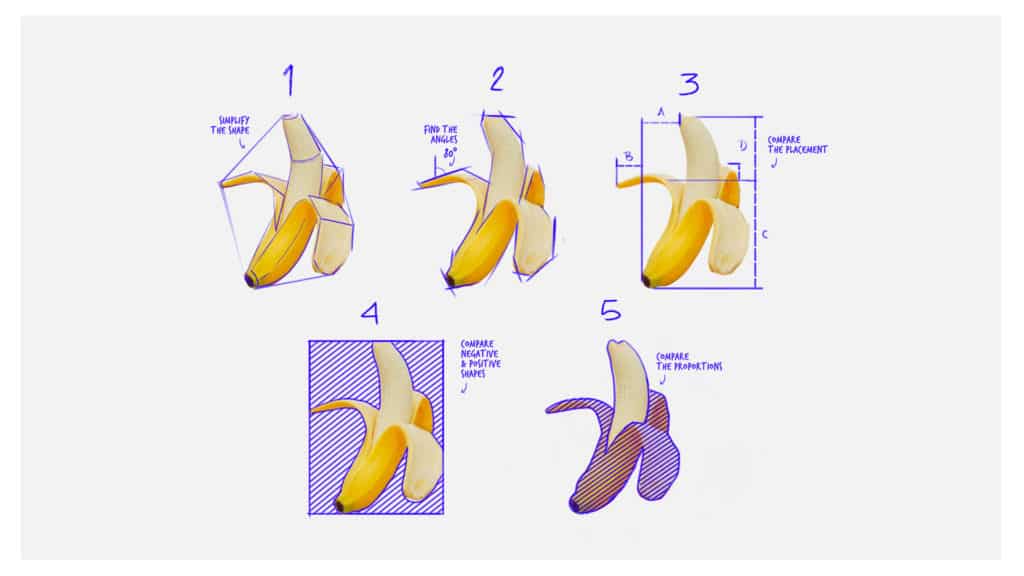The image is an educational illustration demonstrating how to draw a banana in five distinct steps, labeled 1 through 5. Each banana is partly peeled, with the yellow peel pulled back to reveal the cream-colored interior. The bananas are organized in two rows; the top row contains three drawings, while the bottom row holds two. The drawings include a series of straight blue lines, appearing to guide the viewer through the process. Various stages of drawing refinement are present in each illustration, with purple lines tracing key banana features in the early steps and more complex analysis in the latter steps. The detailed instructions and annotations are in blue text, albeit too small to read. The entire illustration is set against a white background, with one of the bananas in step five appearing slightly different in color compared to the others.